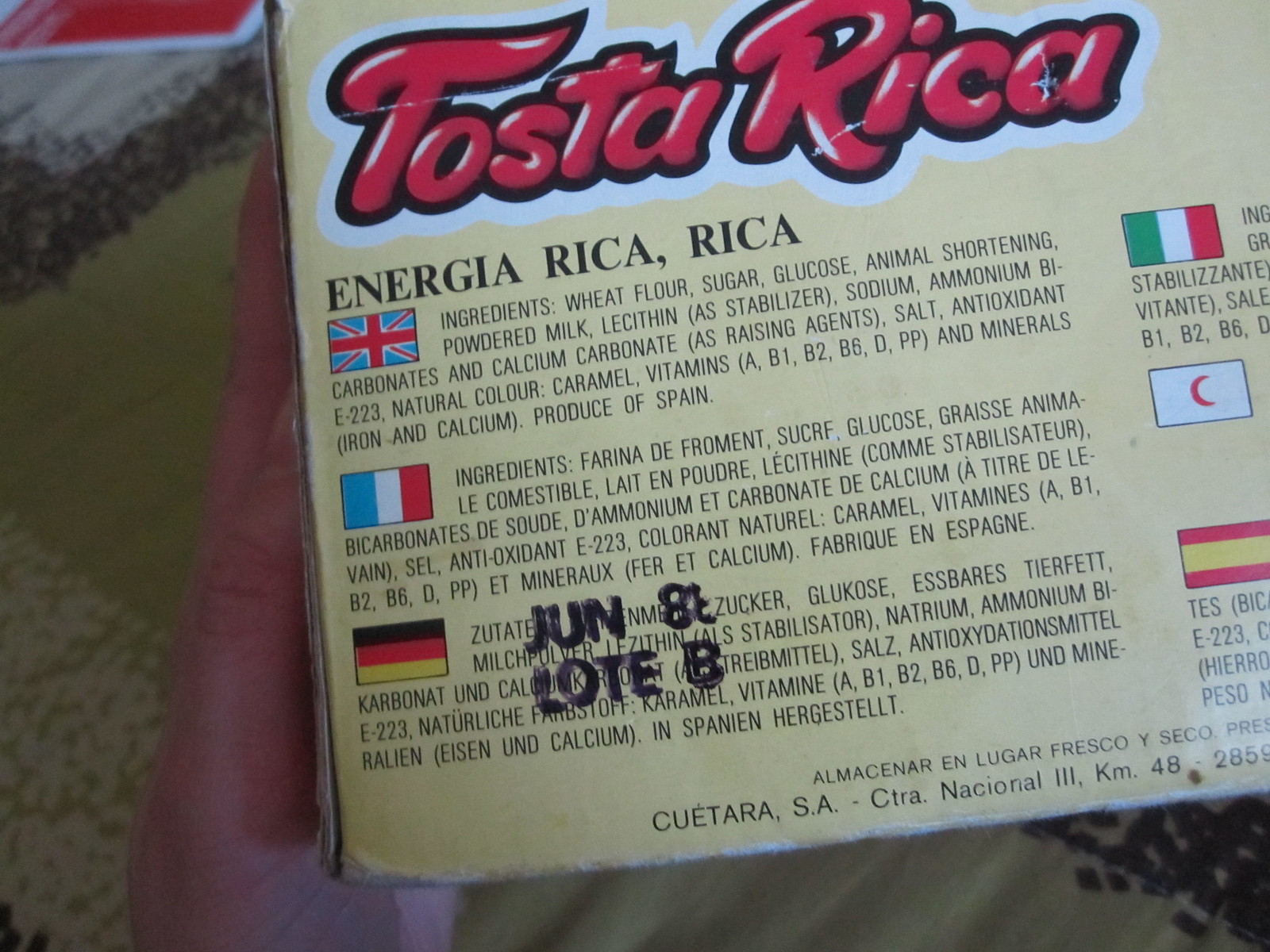The close-up photograph captures the back of a weathered, old cardboard box for a product named "Tosta Rica." The box is held up by an adult hand with white skin, positioned to the left and bottom of the image. The box's top features the brand name "TOSTA RICA" written in bold, stylized red letters with a black outline, reminiscent of graffiti, adding a modern and playful touch. Beneath this, "ENERGIA RICA, RICA" is printed in standard black font.

The ingredients are prominently listed in multiple languages, starting with English, followed by French (accompanied by a French flag icon), German (with a German flag icon), and Italian (flanked by an Italian flag). Two additional flags are visible: one white with a red crescent moon, suggesting it might be from Tunisia, and another yellow with two red bars, indicative of Portugal. The ingredients listed include wheat flour, sugar, glucose, animal shortening, powdered milk, lecithin as a stabilizer, sodium and ammonium bicarbonate, calcium carbonate, salt, antioxidant E223, natural caramel color, vitamins (A, B1, B2, B6, D, PP), and minerals (iron and calcium), denoting a rich and varied composition.

Notably, the packaging suggests the product originates from Spain, bearing the stamp "Produce of Spain." Alongside the multilingual ingredient list, there is a partially smeared black stamp at the lower left reading "J-U-N 8" and "LOTE B." Additionally, there is text in Spanish at the bottom, reading "ALMACENAR EN LUGAR FRESCO Y SECO, CUÉTARA, S.A., CTRA Nacional, 3 KM 48." The box's overall pale yellow hue contrasts with the vibrant lettering and flag icons, enriching its visual appeal and hinting at a long history, as seen by its worn edges.